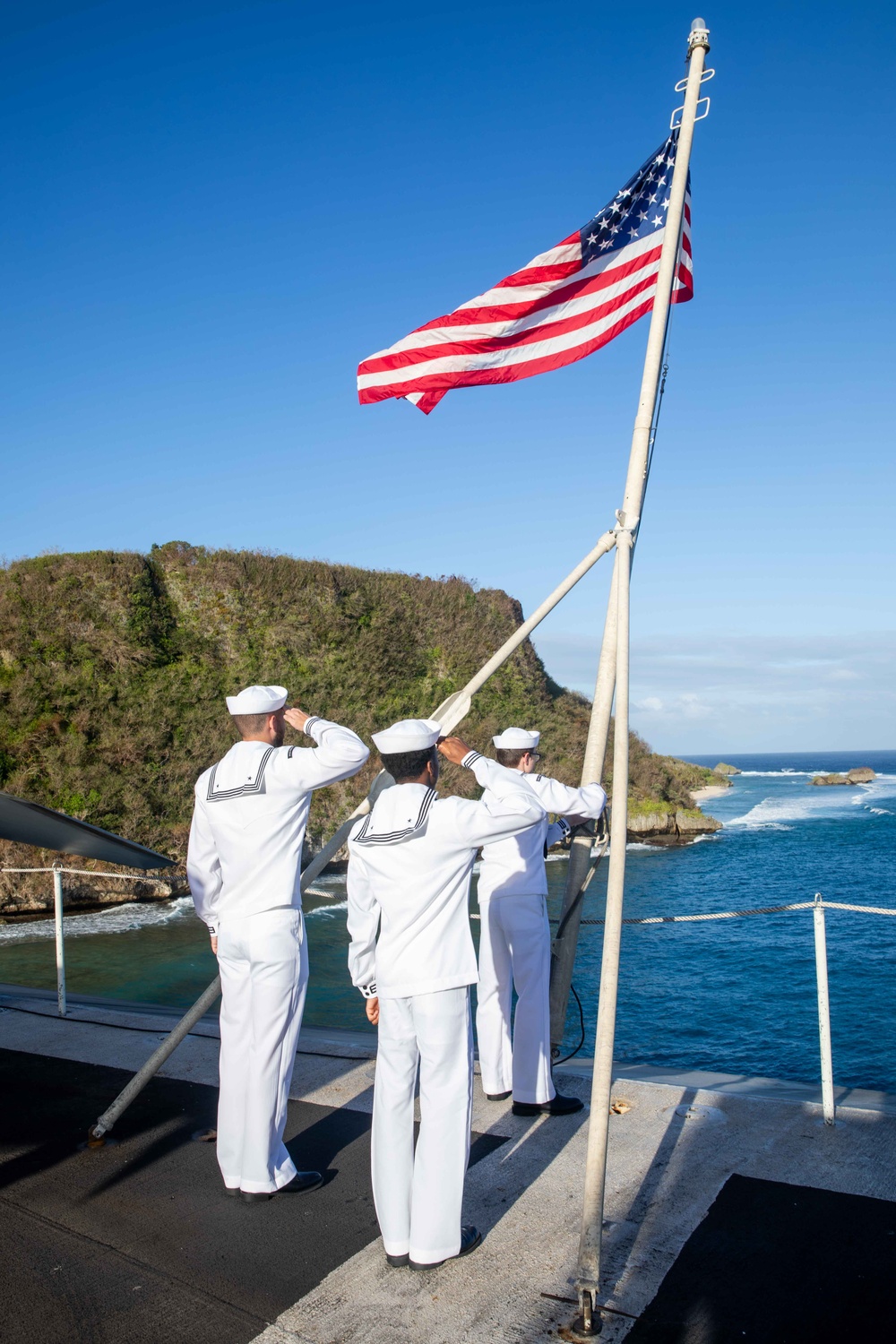In this detailed image, three United States sailors, dressed in traditional white Navy uniforms with square bibs, stand on a pier or possibly the deck of a boat. They face away from the viewer towards the ocean, with a clear blue sky and sparse fading clouds indicating it's likely midday. Two sailors stand in the background saluting, while a third sailor, shorter and younger, hoists an American flag on a pole in the foreground. The flag, slightly folded over itself, points to the left at the top of the flagpole. 

The sailors display a mix of skin tones: a darker-skinned individual on the left and a taller, muscular white-skinned individual. The scene captures a moment of solemn respect as the sailors honor the flag against a backdrop of the vast ocean stretching out to the right, where waves break on the rocks near the coastline. To the left, there is a rocky outcrop covered with low grassy vegetation and a somewhat rocky hill or mountainous range. There is also a metallic wing-like structure in the middle ground left and a rope along the side of the pier or deck where the sailors stand.